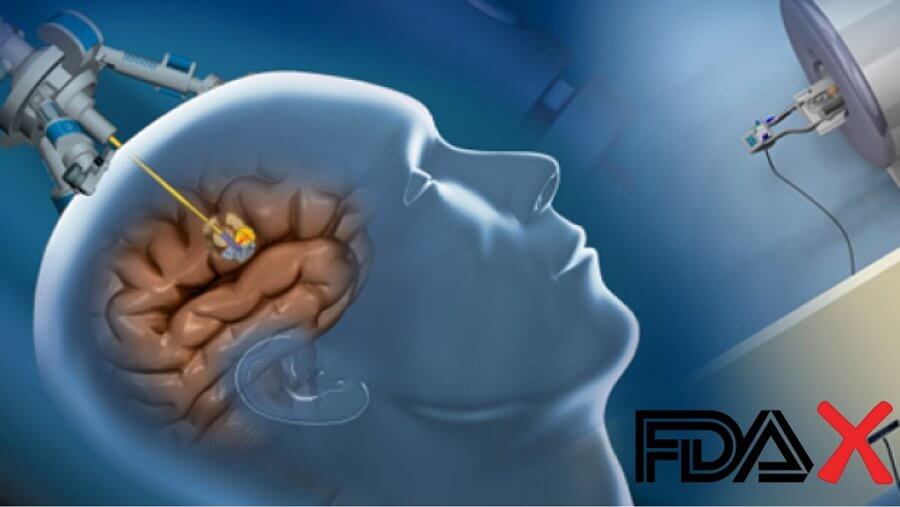The image is a highly detailed, computer-generated 3D illustration depicting a medical procedure. It features a translucent human head, angled and with closed eyes, exposing the internal view of the brain. Over the brain hovers a sophisticated medical device with several nozzles; the central nozzle appears to emit a laser penetrating the skull, simulating a surgical operation. The skin is depicted in a bluish hue, while the brain is rendered in flesh tones. In the bottom right corner, the letters "FDA" are stylized in black, interconnected, and accompanied by a prominent red X. The composition suggests an advertisement for a surgical procedure or medical equipment, emphasizing the technological intricacies and precision involved in the process.